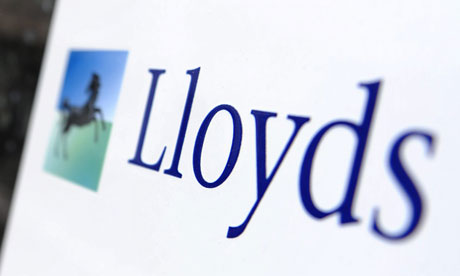This extreme close-up image, likely of a computer screen or poster, features a bright white background with a discernible border suggesting it is confined within a perimeter. On the left side of the image, there's a slightly out-of-focus picture of a black horse that appears to be either jumping or rearing. The sky above the horse is blue, and the bottom portion of the background has light green hues, indicating grass or sand. Next to the horse, in bold navy blue text, is the word "Lloyds" with a capital 'L' followed by lowercase letters. The letters 'L', 'O', and 'Y' are sharply in focus, while the rest transition into a slight blur. This text is indicative of a company logo. The entire layout is slightly diagonal with a subtle light effect on either side, enhancing the image's dynamic appearance.